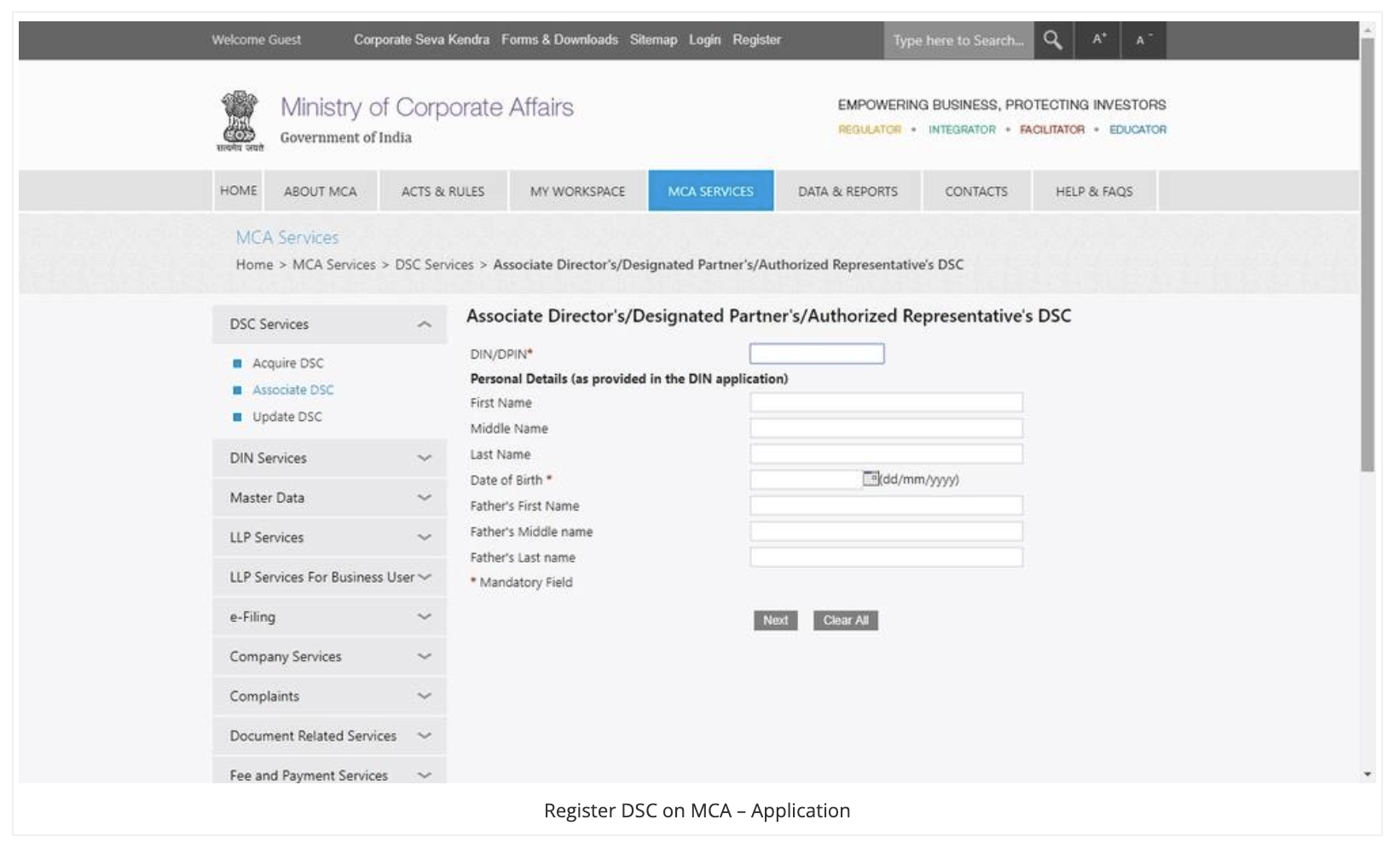**Detailed Caption for the Image:**

The image depicts a comprehensive screenshot of an Indian government website, specifically the Ministry of Corporate Affairs (MCA). At the very top of the website, a long gray bar spans across the page, featuring various navigation options in white text. From left to right, these options include "Welcome Guest," "Corporate Services," "Forms and Downloads," "Sitemap," "Login," and "Register." Adjacent to these links, there's a fainter gray search box labeled "Type Here to Search," accompanied by a white magnifying glass emblem to assist users in finding specific information. To the right of the search box are two black boxes with the letters 'A' and arrows pointing up and down, used for adjusting the text size. On the far right is the scroll bar for navigation.

Below this gray bar, there is a prominent white header with the logo on the left, and in gray letters, the text "Ministry of Corporate Affairs" followed by "Government of India" indicating the website's official nature. Towards the right side of this header, the slogan "Empowering Business, Protecting Investors" is displayed in black letters. Below this, phrases such as "Regulator" in orange, "Integrator" (though partly illegible) in blue, and "Facilitator" in red further describe the entity's roles, accompanied by another slogan, "Educator."

Beneath this main header is a detailed gray navigation bar with clickable menu options in black letters. These options read from left to right: "Home," "About MCA," "Acts and Rules," "My Workspace," the highlighted "MCA Services" in blue with white letters, "Data and Reports," "Contacts," "Help," and "FAQs." Below this, another gray bar provides breadcrumb navigation in faint blue letters with "MCA SERVICES" in red, creating a seamless user pathway through "Home > MCA Services > DSC Services > Associate Directors / Designated Partners / Authorized Representatives."

In the central portion of the webpage, large black text labels the section for "Associate Directors / Designated Partners / Authorized Representatives (DSC)." This area features multiple text boxes for data entry, allowing users to fill in information like "DIN / DPIN (required)," personal details (as per DIN application), "First Name," "Middle Name," "Last Name," "Date of Birth (required)," and "Father's Name." Each field is accompanied by a red asterisk for mandatory fields, and there's a calendar icon next to the date of birth field for correct date entry. At the bottom of the form, two gray buttons are available: "Next" in white letters on the right and "Clear All" on the left.

On the left side of the main content, there's a tall gray menu with the heading "DSC Services" and an upward-pointing V. Below this heading are options with blue squares: "Acquire DSC," "Associate DSC," and "Update DSC," all in capital letters. Following these options are additional categories in gray boxes with dropdown arrows indicating further selections: "DIN Services," "Master Data," "LLP Services," "LLP Services for Business User," "e-filing," "Company Services," "Complaints," "Document Related Services," and "Fee and Payment Services." Finally, there is a black text prompt for "Register DSC on MCA Application."

The image captures a structured and user-friendly layout designed for efficient navigation and form completion, confirming its identity as a sophisticated digital interface for the Ministry of Corporate Affairs in India.